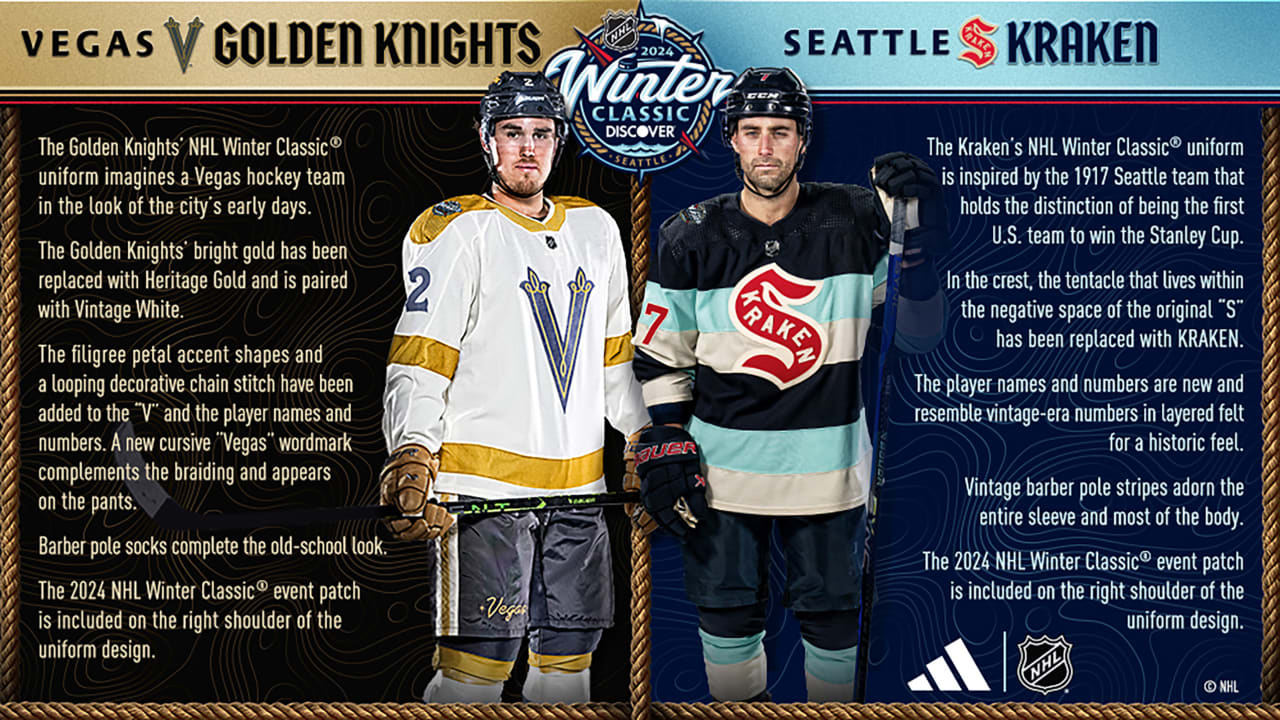This detailed poster advertises the 2024 Discover Winter Classic, showcasing a highly anticipated hockey match between the Vegas Golden Knights and the Seattle Kraken. On the left side, player number two of the Vegas Golden Knights stands prominently, sporting a vintage-inspired uniform. This design, rooted in the aesthetics of Las Vegas' early days, features heritage gold in place of bright gold, combined with vintage white. Notable details include gold trim along the sleeves, waist, and shoulders, with the vintage touch highlighted by fleece accent petal shapes and loops reminiscent of old-school styles.

Opposite him, player number seven of the Seattle Kraken is depicted, clad in a uniform paying tribute to the historic 1917 Seattle team, the first U.S. team to win the Stanley Cup. This design includes a distinctive crest featuring a tentacle, symbolizing the Kraken. The uniform combines classic elements like barber-style pull socks, with modern touches such as wing-inspired player names. Both players stand side by side, providing a striking comparison of the unique, historically-inspired uniforms set against detailed background descriptions that highlight the historical and cultural inspirations behind their designs.